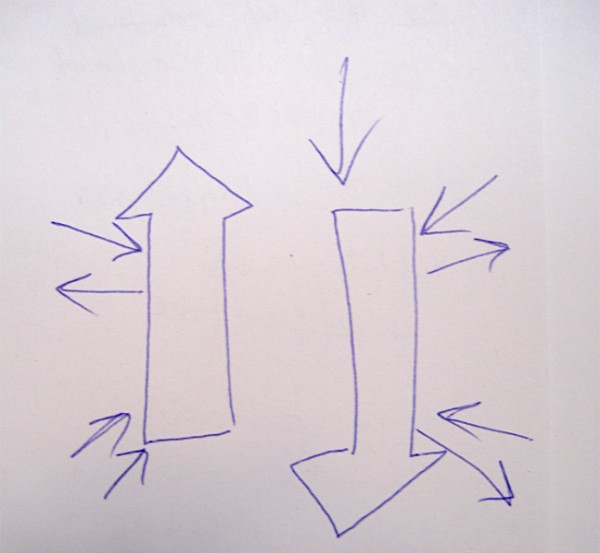The drawing features a series of arrows rendered in blue pen ink. The composition is dominated by two large, bold arrows: one on the left pointing upward, and one on the right pointing downward. Surrounding these dominant arrows are smaller, less detailed arrows. These smaller arrows are predominantly paired and are situated on the perimeter of the large arrows but do not occupy the space directly between them.

The upward-pointing arrow has four smaller arrows: three are directed inward towards the larger arrow, while one points outward. In contrast, the downward-pointing arrow is accompanied by five smaller arrows: three directed inward and two directed outward. Despite the presence of these smaller arrows, there is an absence of a discernible pattern to their arrangement, creating a seemingly random but paired structure with one pairing exception.

Overall, the intricate network of arrows presents a visually compelling arrangement where the large arrows create a focal point, and the smaller arrows add complexity and nuance to the design.